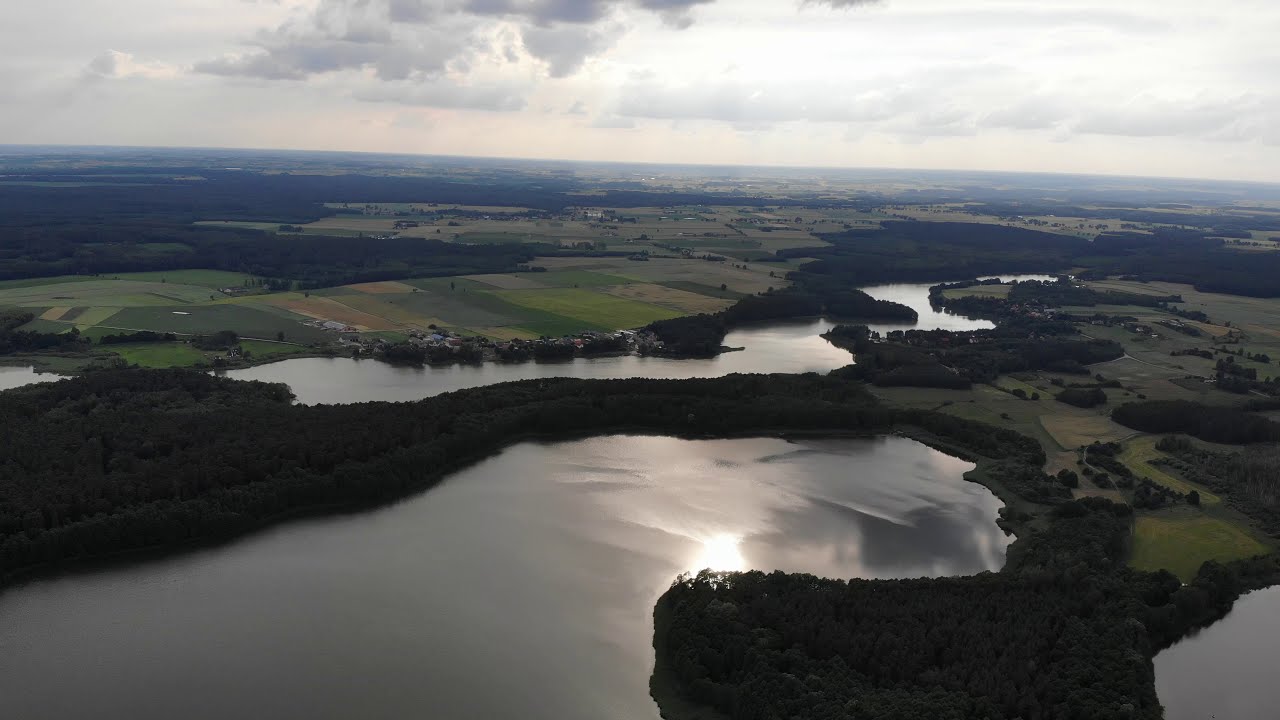This aerial view captures a serene countryside landscape featuring a centrally positioned lake surrounded by lush, dark green trees and interspersed open fields of green, brown, and tan hues. Along the horizon, a foggy and overcast sky occupies the top quarter of the image, with white and gray clouds adding a muted, dreary ambiance. Small, barely discernible homes dot the landscape near the lake, blending into the environment. A twisting river curves in an S-pattern beyond the lake, also enveloped by dense tree canopies. The flat, still water surfaces reflect the sunlight, contrasting with the almost black appearance of the trees, emphasizing the calm yet intricate beauty of this countryside tableau.